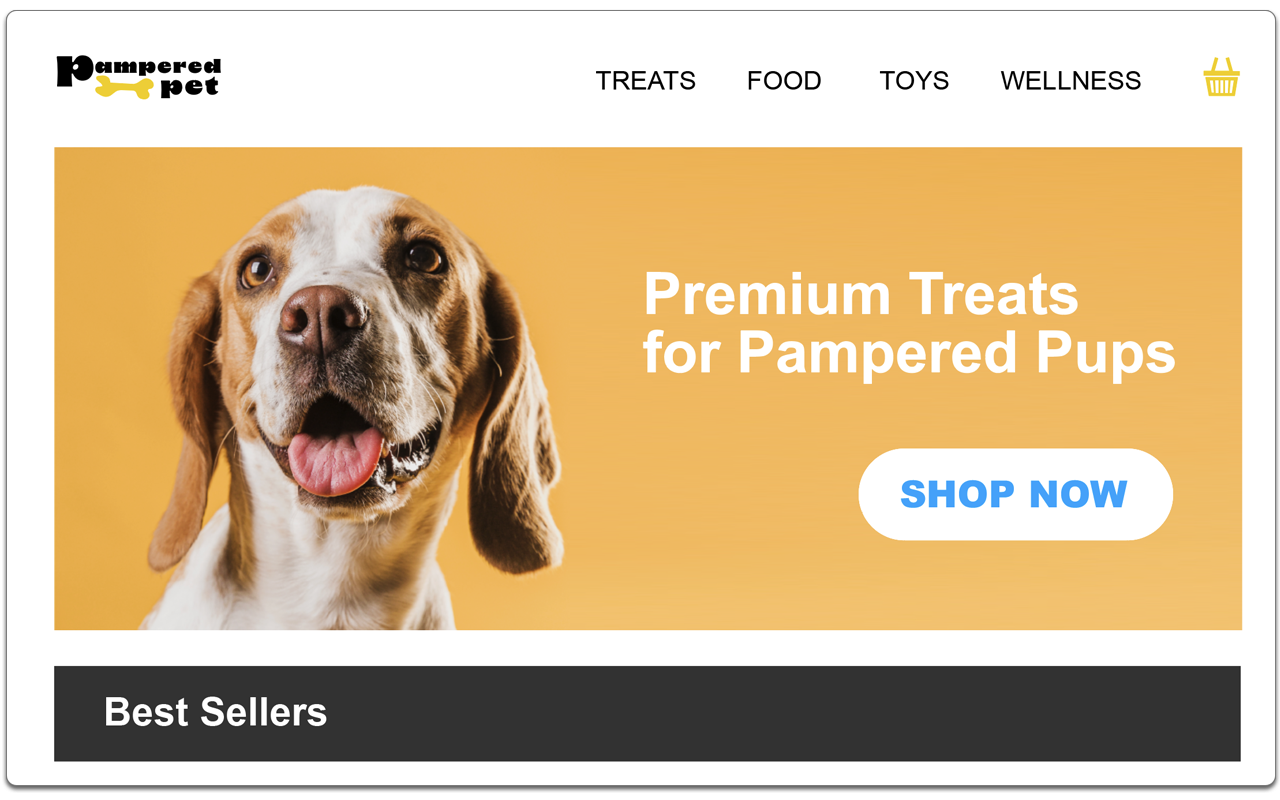Screenshot of the "Pampered Pet" webpage featuring a white background with the title "Pampered Pet" in black letters located in the upper left corner, accompanied by a yellow dog bone graphic. In the upper right corner, there are categories listed: "Treats," "Food," "Toys," and "Wellness," followed by a shopping cart icon.

The center of the page is dominated by a large orange rectangular box showcasing a close-up image of a beagle. The beagle, predominantly white, has distinct brown markings around and below its eyes, which extend to its cheeks, and light brown, floppy ears. The dog’s eyes and nose are dark brown, with a small patch of black fur under the nose. The beagle's tongue, pink and slightly dry, is sticking out, and its mouth appears wet on one side.

To the right of the beagle’s image, the text reads "Premium Treats for Pampered Pups." Below this text is a white oval-shaped button with blue writing that says "Shop Now." At the bottom of the page, there is a long black bar labeled "Bestsellers."